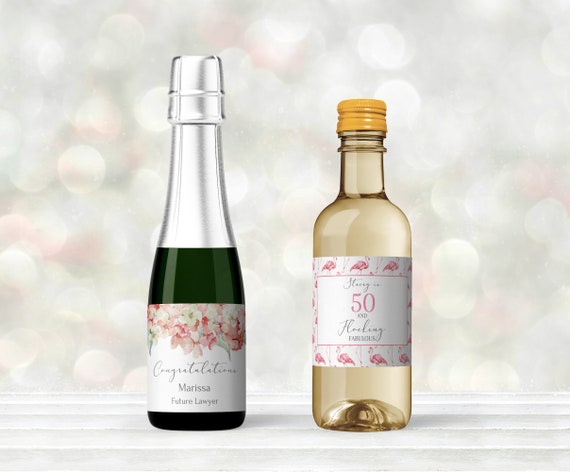The photograph showcases two small travel-sized wine bottles, centrally positioned, likely intended for a retailer's website or as celebratory party favors. The bottle on the left stands slightly taller, adorned with a silver foil top and a dark green glass base. Its label is detailed with an array of white and pink flowers, accented by green leaves, and features the cursive inscription, "Congratulations, Marissa, Future Lawyer," against a white background. The bottle on the right, slightly shorter and shaped like a traditional nipper, has a yellow-tinted glass with an orangish cap. It carries a large white label bordered by repeated illustrations of pink flamingos. Prominently displayed in the middle of this label is the number "50" in pink, although the surrounding text is indistinct. The bottles rest on a surface resembling white wooden slats, horizontally arranged, with an artistic backdrop of out-of-focus, colorful, circular lights that add a festive ambiance to the scene.